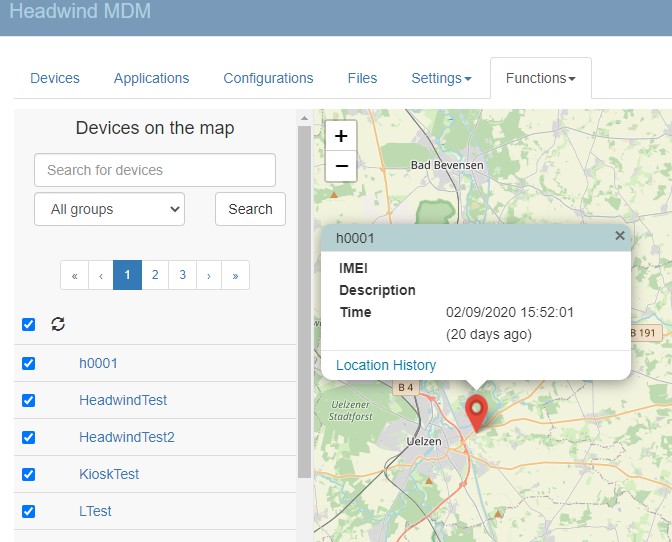The image portrays a detailed map interface from the Hedwin MDM (Mobile Device Management) system. The interface has a clean, off-grey, pale blue top border that contains various menu tabs, including Devices, Applications, Configurations, Files, Settings, and the currently selected Functions tab.

The main content area of the interface is divided into two sections. On the left, a panel is dedicated to devices on the map. It includes a search field, a drop-down menu labeled "All Groups," and a search button. Below these elements, pagination controls allow navigation through device pages, featuring double left-facing arrows, a left-facing arrow, page numbers one through three, a right-facing arrow, and double right-facing arrows. A list of devices is displayed below these controls, each with a checkbox. The devices listed are H0001, Hedwin test, Hedwin test two, kiosk test, and L test, with a refresh symbol at the top.

The right section of the interface displays the map itself. There are controls available to adjust the map size. A pop-up box is centrally located over a map marker, labeled with H0001. Within this pop-up, detailed device information is presented, including the IMEI, description, timestamp of 15:52:01 on 02-09-2020, and a note indicating that this was 20 days ago. The bottom part of the pop-up contains an option to view the device's location history.